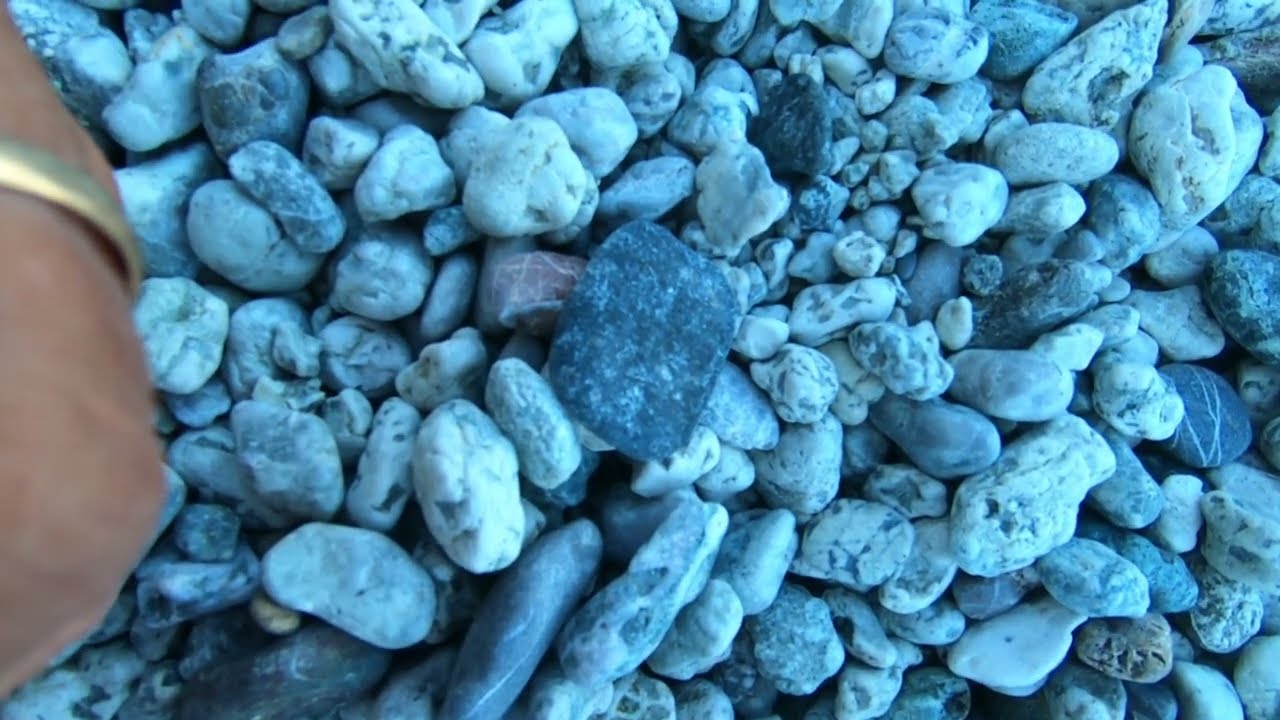The image captures a close-up scene dominated by various rocks illuminated with heavy blue lighting. The rocks, mostly white with gray speckles, vary in different shapes and sizes, ranging from smaller than a knuckle to approximately the same size as a knuckle. Among these, a prominent rectangular black rock with white speckles stands out in the center. Below it lies a tan-colored rock. On the left side of the image, a large light-skinned human finger adorned with a simple gold ring is visible, suggesting the human scale and interaction with the scene. The rocks appear mostly smooth with occasional pits, layered in such a way that they form a solid mass. The overall blue hue and close-up perspective give a surreal, almost underwater appearance to the collection of small pebbles.